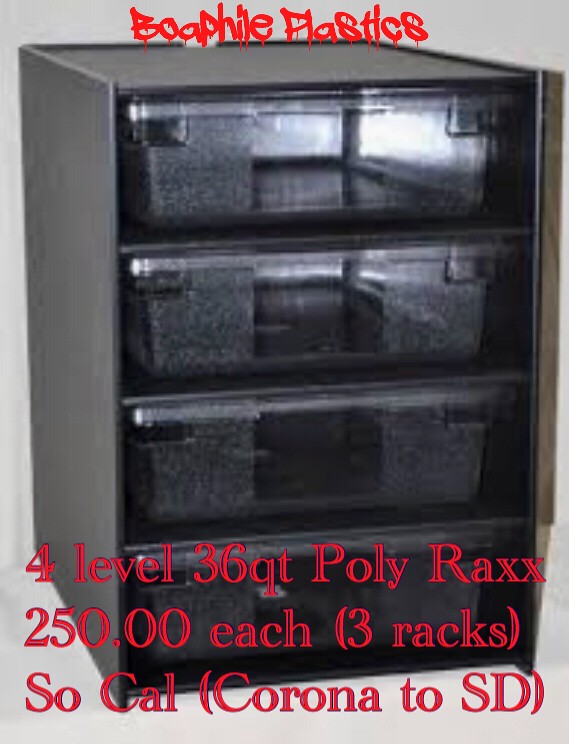The image depicts a set of black, stackable plastic storage containers, organized into a four-tier shelving unit. Each of the four levels features a pull-out bin, and the unit is encased within a larger rectangular frame. At the top of the shelving unit, red cursive or "dripping" text reads "Boophile Plastics." Below, additional text in a different shade of red specifies, "4 Level 36 QT Poly Racks, $250.00 each, 3 Racks (SoCal, Corona to SD)." The background is predominantly white, giving the image an impression of the unit floating without any visible support.